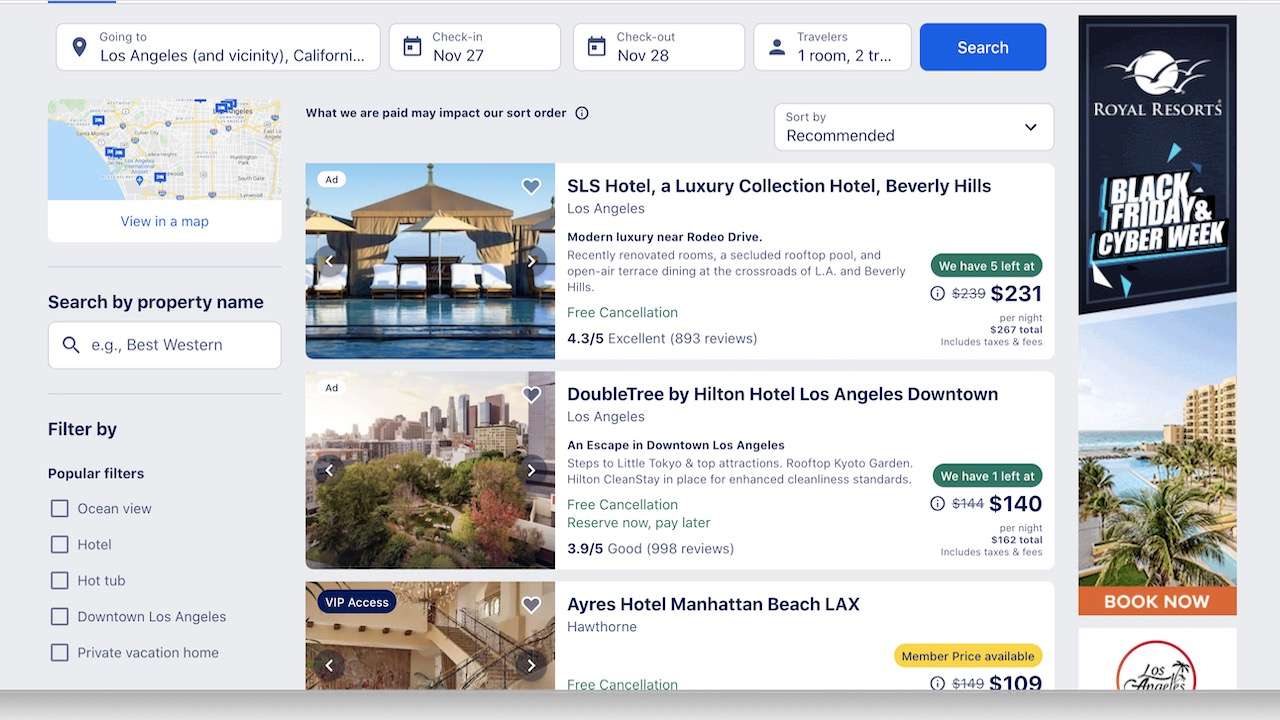This screenshot captures a comprehensive overview of a travel booking website interface aimed at planning a trip to Los Angeles. The browser's address bar, browser type, and operating system are not visible, placing full attention on the website's features from left to right.

On the top-left corner, a mini map pin indicates the destination, "Los Angeles and vicinity, California." A calendar icon shows the booking dates: check-in on November 27th and check-out on November 28th. Travelers details suggest one room, likely for two travelers, though this information is cut off. A prominent "Search" button in white text on a blue rectangle invites users to find available accommodations.

Adjacent to this, users have options to view properties on a map, search by property name (with a magnifying glass icon, e.g., Best Western), or apply popular filters like "ocean view," "hotel," "hot tub," "downtown Los Angeles," and "private vacation home."

On the right side, a couple of advertisements catch the eye: one for Royal Resorts showcasing a flock of seagulls with "Black Friday and Cyber Week" deals in white text, and another depicting a seaside hotel, encouraging viewers to "book now" in white text on an orange background. The bottom half of this ad is cut off, showing only "Los Angeles."

A small disclaimer informs that payment from properties may affect their order of appearance. The listings are sorted by "recommended" and feature sponsored results marked with hearts.

Highlighted properties include:
1. **SLS Hotel, a Luxury Collection Hotel, Beverly Hills, Los Angeles**: This modern luxury hotel is near Rodeo Drive, offering renovated rooms, a secluded rooftop pool, and open-air terrace dining. It boasts a rating of 4.3 out of 5 from 893 reviews, with free cancellation. Only 5 rooms are left, priced at $231 per night (down from $239), totaling $267 including taxes and fees.

2. **DoubleTree by Hilton Hotel, Los Angeles Downtown**: Located in downtown LA, this hotel is close to Little Tokyo and key attractions, featuring a rooftop Kyoto Garden and adhering to enhanced cleanliness standards. It has a rating of 3.9 out of 5 from 998 reviews, with free cancellation and a "reserve now, pay later" option. Only 1 room is left, priced at $140 per night (down from $144), totaling $162 including taxes and fees.

3. **Ayers Hotel Manhattan Beach, LAX, Hawthorne**: Highlighted as "VIP Access," this hotel offers free cancellation and a special member price of $109, reduced from $149.

The website user appears to be planning a trip to Los Angeles, searching for upscale accommodations in desirable locations.